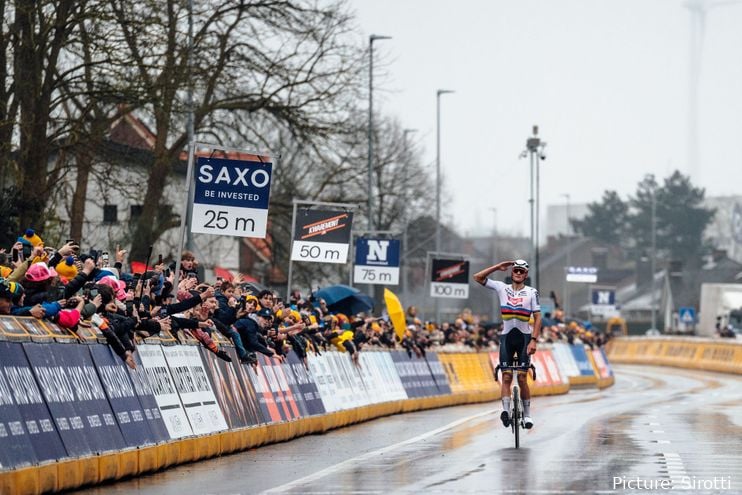In this vivid color photograph, we observe a cyclist participating in a race, riding a bicycle on a wet road surface. The cyclist, dressed in dark shorts and a white top adorned with blue, red, and yellow stripes across the chest, also sports a white helmet and dark sunglasses. He is seen saluting the crowd as he stands up on his bike, his right hand raised to his forehead. The road is wet, indicating recent or ongoing rain, and the sky overhead is dark and overcast, creating a dreary atmosphere.

On the left side of the image, a substantial crowd of spectators is gathered behind barriers, cheering on the cyclist. The barriers are adorned with various blue, orange, and yellow advertisements, along with flagpoles displaying assorted signs. Notably, the signs read 25M, 50M, 75M, and 100M, marking the race distances. In the background, we see bare trees and a white building with a brown or red roof, which adds to the whole scene's muted color palette.

The right-hand side features a solid yellow barrier with illegible text. Additionally, trees are visible on both sides of the scene, lining the race track. At the bottom right corner of the image, the words "Picture Siradi" are inscribed in white letters. Despite the overcast conditions, the natural daylight provides sufficient clarity for the outdoor setting, ensuring that all aspects of the race and the environment are clearly visible.